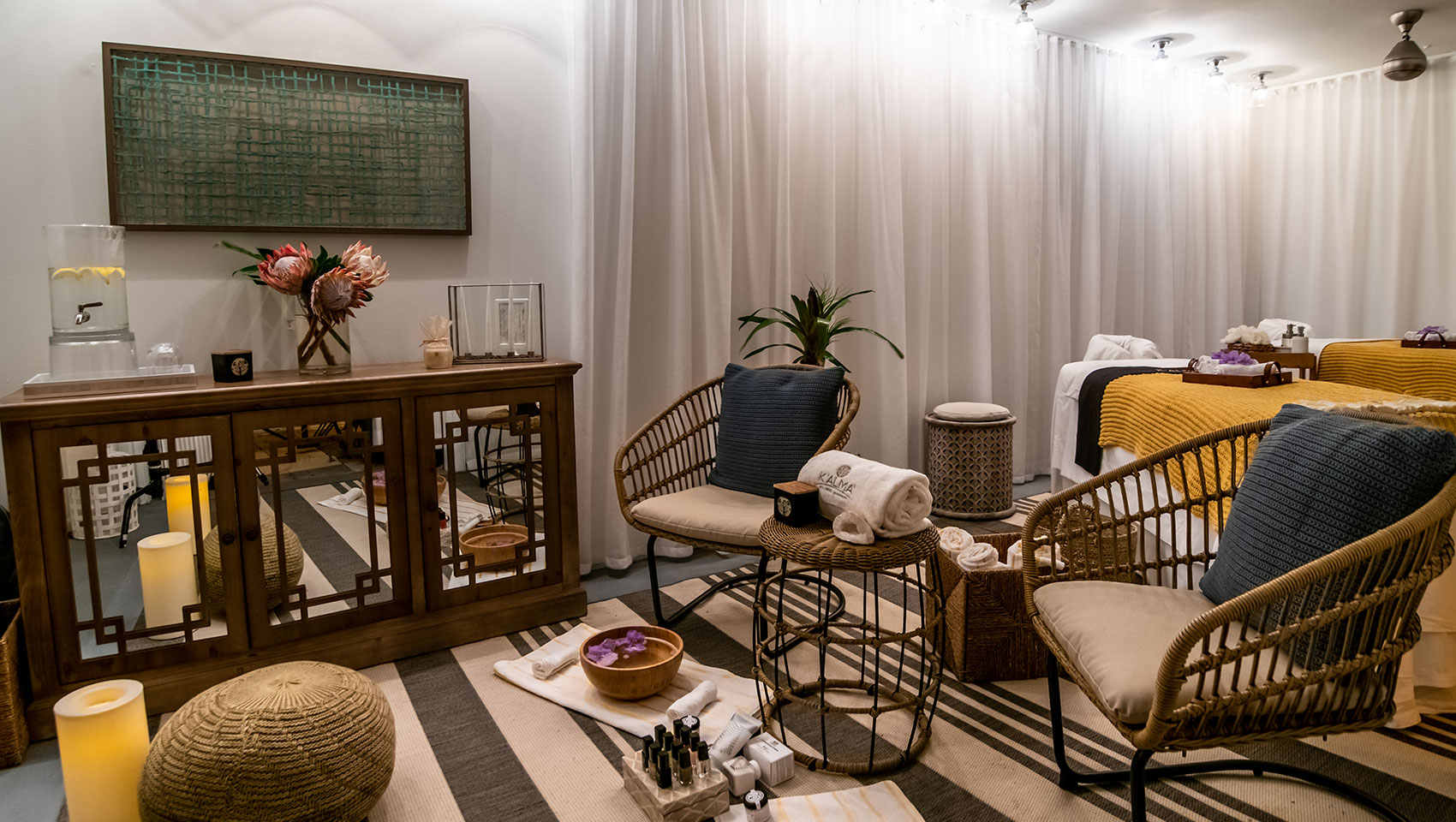This image depicts a serene, well-decorated massage room, designed for a calming experience, possibly accommodating couples massages or dual treatments. Dominating the right side of the room are two massage tables, each draped with yellow blankets and prepared with essential oils, indicating the space's readiness for its next clients. The central area features wicker furniture, including two chairs fitted with white cushions and blue pillows, and a small wicker table between them, holding a rolled towel and a small decorative box. A woven basket with additional rolled towels sits nearby.

The floor is covered with a tan carpet, extending across the majority of the room, adding to the overall warmth of the decor. The walls are adorned with slightly off-white curtains, enhancing the room's tranquil atmosphere. To the left, a low mirrored cabinet holds various items: a vase with three pinkish-red flowers, a pitcher of lemon water, a frame, and some candles. Mounted above the cabinet is a rectangular artwork featuring strings stretched in a grid-like pattern.

Additionally, a wooden bowl filled with water and floating petals is positioned below the wicker chairs, suggesting the availability of pedicure services alongside massages. This room exudes an inviting and peaceful ambiance, perfect for relaxation and rejuvenation.